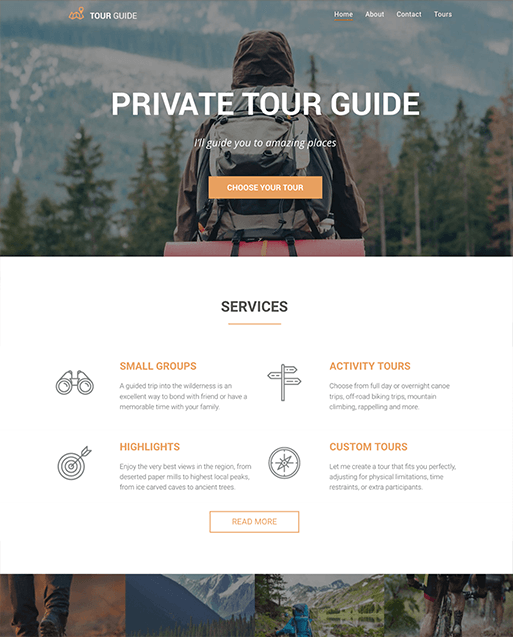This is a detailed screenshot of a landing page from "Tour Guide." The logo, which consists of an orange map with a location dot, is prominently displayed at the top left corner. On the top right side, there's a menu bar with the options: Home, About, Contact, and Tours.

The upper section of the webpage features a captivating background photo of a vast wilderness, including dense trees and towering mountains. In the foreground of this scene, a person, viewed from the back, stands facing the natural splendor, equipped with a backpack, embodying the spirit of adventure.

Overlaying the image, bold text declares "Private Tour Guide," accompanied by a smaller, italicized white text that reads, "I'll guide you to amazing places." Below this inspiring message, an attention-grabbing orange button invites users to "Choose Your Tour."

Transitioning from the image, the background turns to crisp white, where the word "Services" appears centrally in black letters and is underlined in orange. The services section is organized into four distinct categories, each represented by an orange title in all caps, accompanied by a relevant icon and a brief description. From left to right, the categories are: "Small Groups," "Activity Tours," "Highlights," and "Custom Tours."

At the bottom center of this section, a "Read More" button is available, enticing users to explore further. Additionally, there is a slider displaying four images from various tours; however, only a portion of the slider is visible in the screenshot.